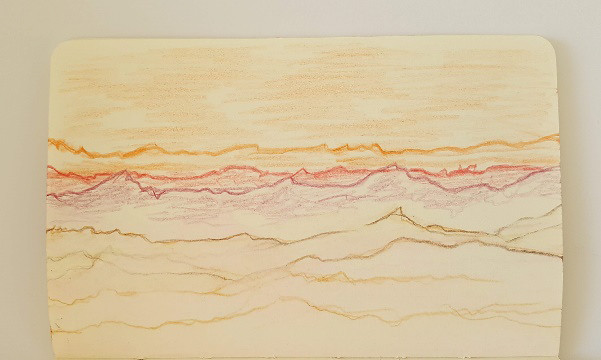The photograph features a horizontally oriented, very large piece of sketch paper with rounded edges, leaning against a white wall. The artwork appears to be created using a combination of crayons, colored pencils, and possibly watercolor pencils or wash. The composition is an abstract landscape with vivid horizontal shading and jagged lines in various colors. 

At the top of the image, wide light pencil strokes in orange suggest an expansive sky. Directly beneath the sky, an irregular, jagged line in dark orange delineates what looks like a mountain range, shaded in orange. Following this, there are successive layers of jagged lines in red, purple, and brown, each suggesting additional mountain ranges or rock formations. These colors continue horizontally shading down the paper in thicker gradations. The bottom section of the artwork features what resembles brown and yellow sand dunes, evoking either a rocky terrain or the sea with wave-like crests. The detailed gradations of color and texture combine to give the abstract landscape a dynamic and multi-layered appearance.